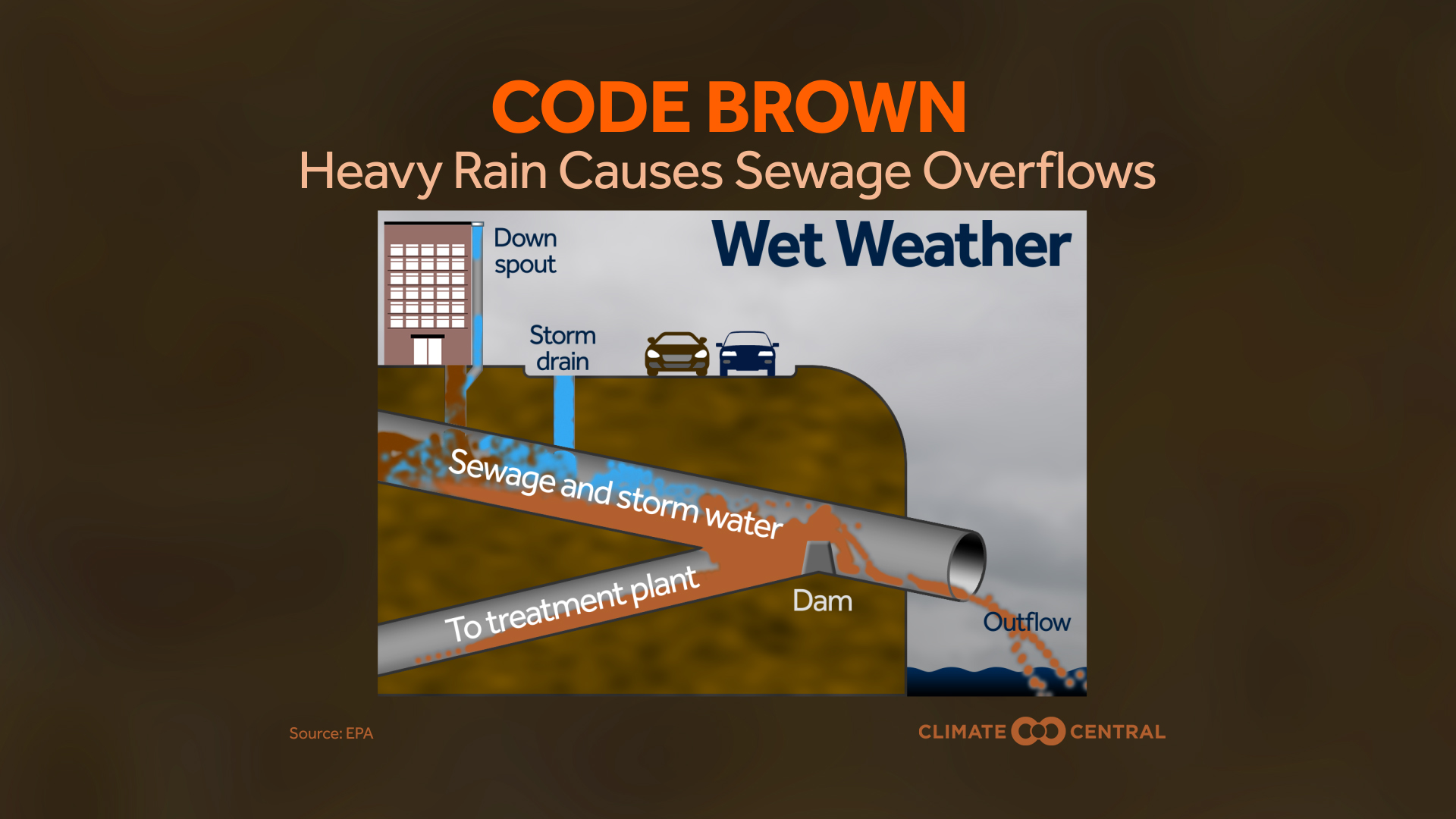This is a detailed infographic depicting the impact of heavy rain on sewage systems against a dark brown background. At the top, orange text announces "Code Brown," with paler light orange text below it reading, "Heavy rain causes sewage overflows." In the lower left, the source is cited as EPA in orange text, and in the lower right, the logo of Climate Central is featured, combining the two C's of the words.

The central illustration shows a simplified diagram of the process. On the upper left, there's a brown building with blue-labeled downspout, connected to a storm drain. The diagram highlights the pipes beneath the ground, including a blue stormwater pipe and a sewage pipe labeled "sewage and stormwater" in white text. These converge and flow towards a middle section featuring a small dam, indicated by "dam" in white text, which blocks part of the flow. Below the dam, a pipe labeled "to treatment plant" directs some of the overflow downwards. When the dam overflows, excess water follows a pipe labeled "outflow" leading to a body of water on the right side of the image. The inset on the diagram depicts a blue sky, two cars on a hill, and the blue-labeled "wet weather" to signify rainy conditions contributing to the overflow.